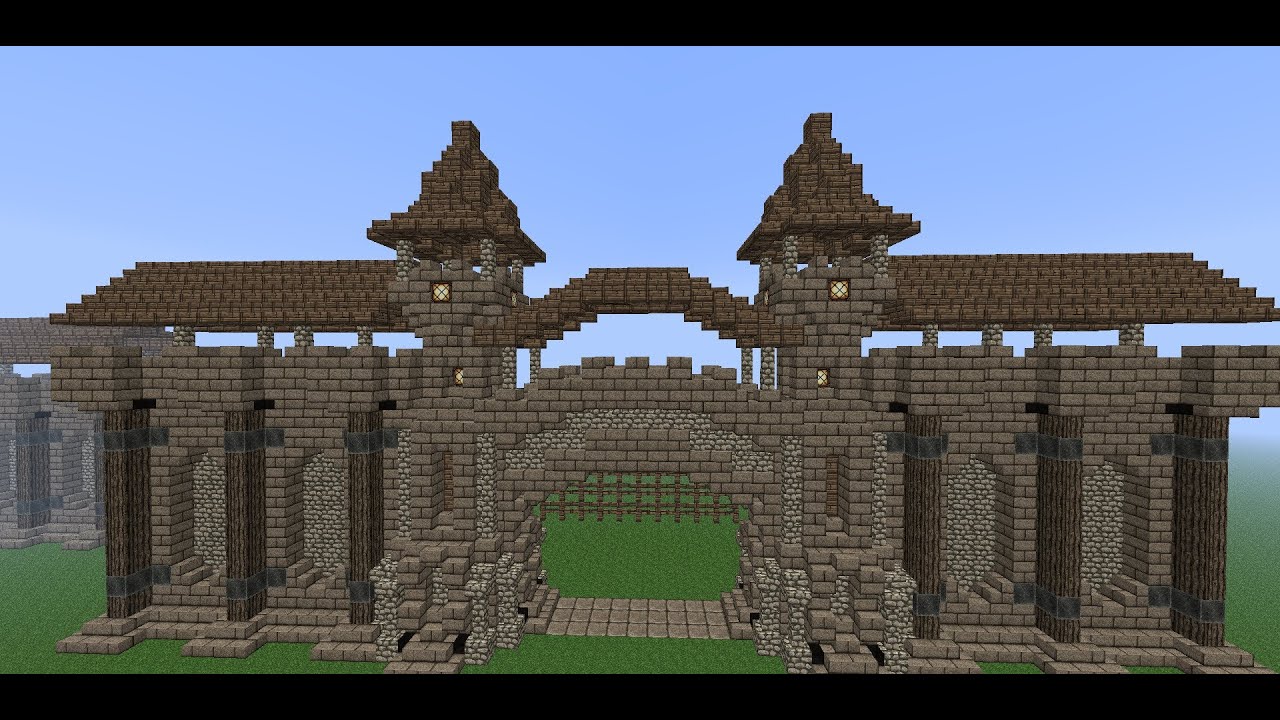This image showcases a highly detailed and meticulously crafted Minecraft structure resembling the front of a medieval castle. The castle façade features a prominently raised portcullis in the center, flanked by two symmetrical towers akin to those found in Harry Potter. The structure is comprised of numerous blocks, each displaying different textures, including cobblestone, stone bricks, wood, and roofing tiles, adding to its intricate design. The columns and arches on either side of the portcullis give it a grand appearance, with pathways running across the top of the gate and extending to the towers on both sides. The castle sits upon a basic green Minecraft grass landscape, with a clear blue sky in the background, underscoring the game's distinctive blocky aesthetic. Additionally, glowstone blocks are used for lighting within the towers, enhancing the castle's medieval ambiance. Overall, this impressive build exemplifies the dedication and skill of its creator, showcasing a blend of artistic vision and detailed craftsmanship.